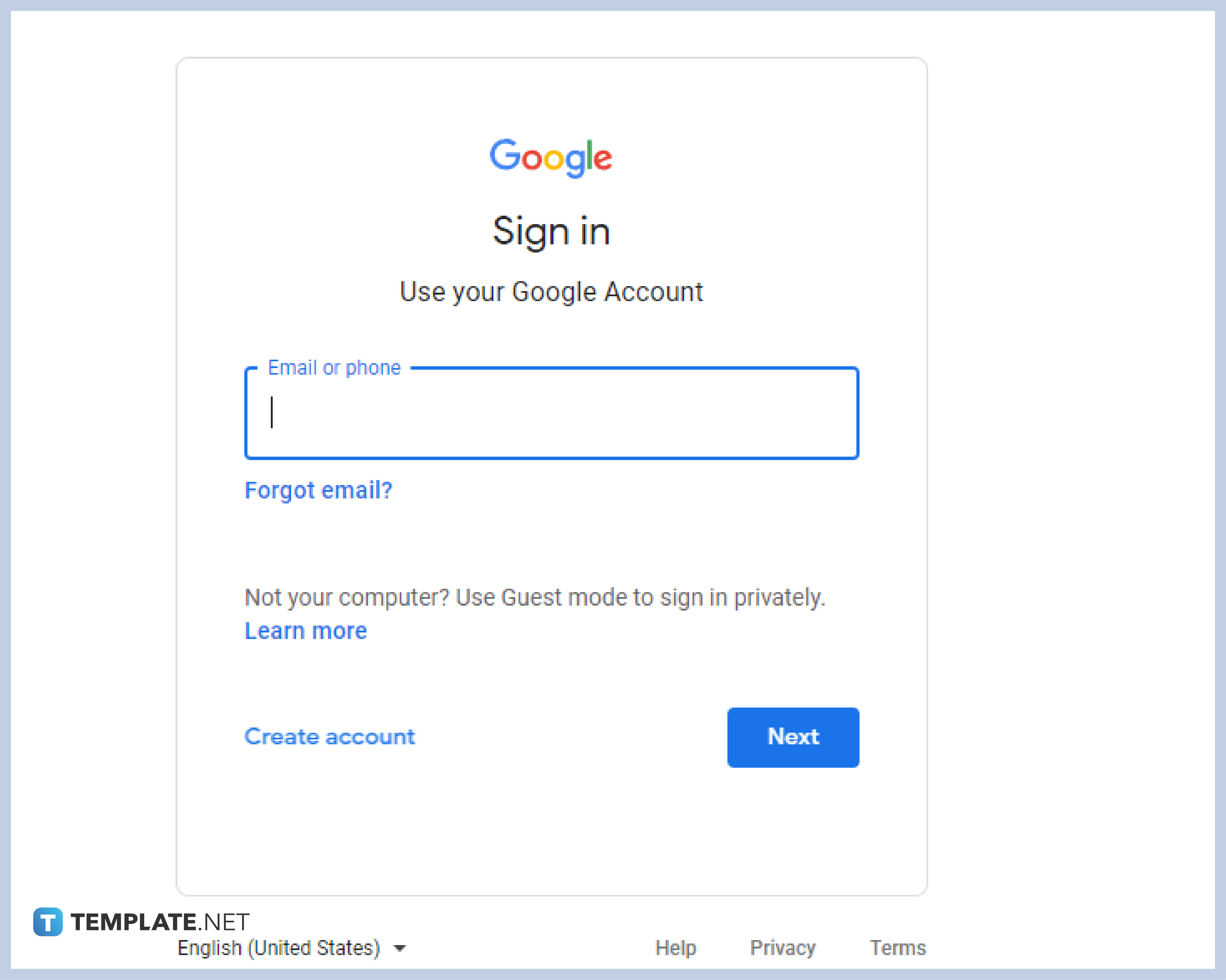This is a screenshot of a Google desktop application's sign-in page. The predominant background is white, overlaid by a grey box outline. At the top of this box, the colorful Google logo is prominently displayed, featuring a capital "G." Below the logo, the text reads "Sign in" and "Use your Google Account."

A long, blue horizontal box is provided for entering an email or phone number, labeled "Email or phone." A text input field is present, with a contextual note indicating that it is ready for user input. Directly below this input field is a blue hyperlink reading "Forgot email?"

Further down, a message in grey text advises, "Not your computer? Use Guest mode to sign in privately," followed by another blue hyperlink stating "Learn more." An option to "Create account" is available as a blue hyperlink as well.

On the right side of the form is a blue "Next" button with white lettering, facilitating progression to the next step. 

At the bottom of the screenshot, a footer bar is visible, containing the text "template.net," "English (United States)" with a drop-down button, and a logo featuring a stylized white "T" inside a blue square. The footer also includes links for "Help," "Privacy," and "Terms" in grey text.